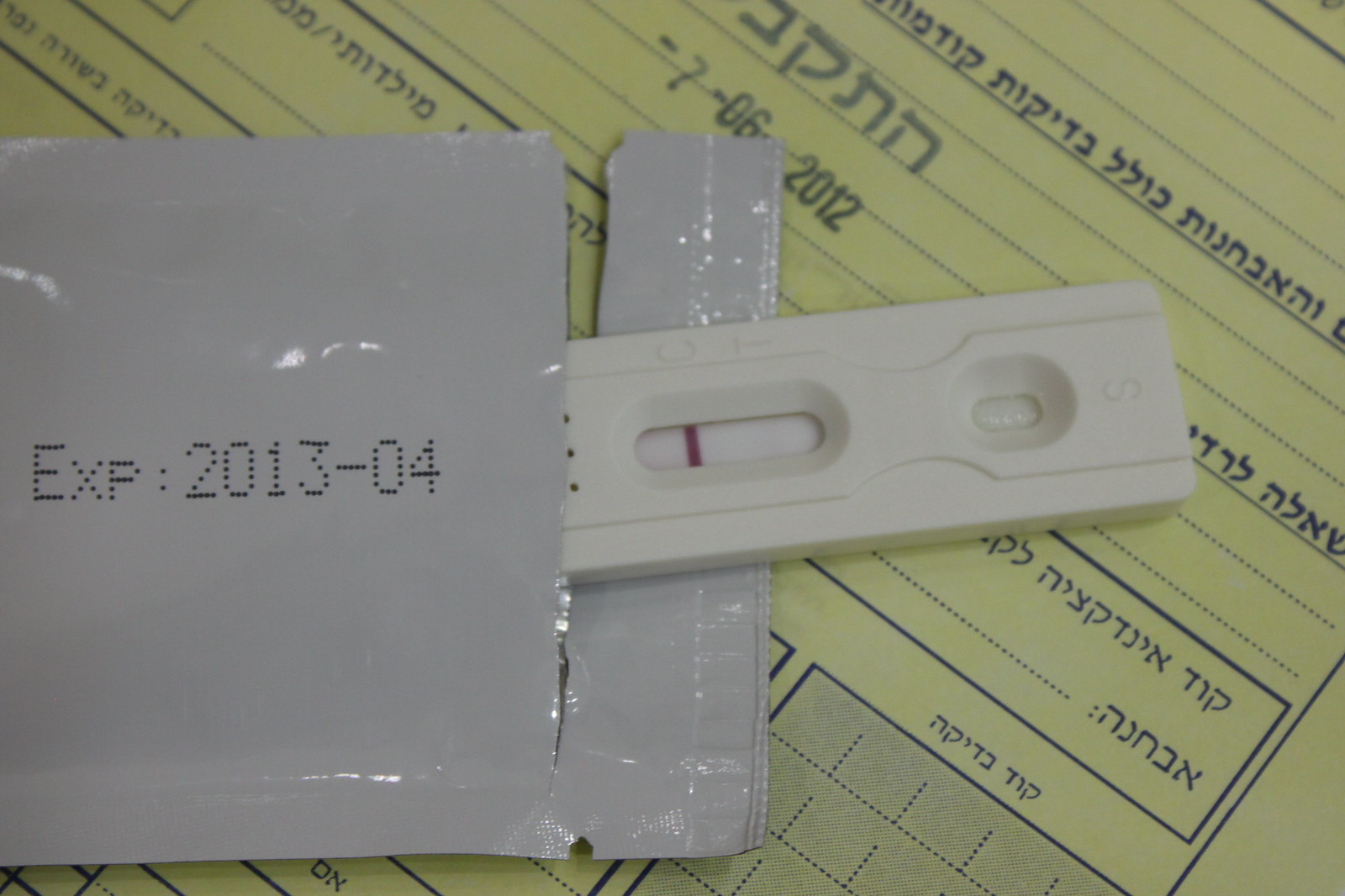The image features a document with a green background, accented by black and gray elements. The document is covered with lines and writing, predominantly in Hebrew. Towards the bottom of the document, there are areas shaded in gray adorned with black dots and lines. At the top, a partial sequence of numbers and a dash can be seen, reading “-7-06...” followed by some obstruction, and then continuing with “2012.” 

There is an open gray packet also visible on the document. The packet is labeled with an expiration date formatted as “exp...2013-04.” Emerging from the packet is a white rectangular item with lined patterns, which seems to have a red line and rounded corners. The rest of the package is visible beneath this item, and just beyond the edge of the packet, three black dots are noticeable.